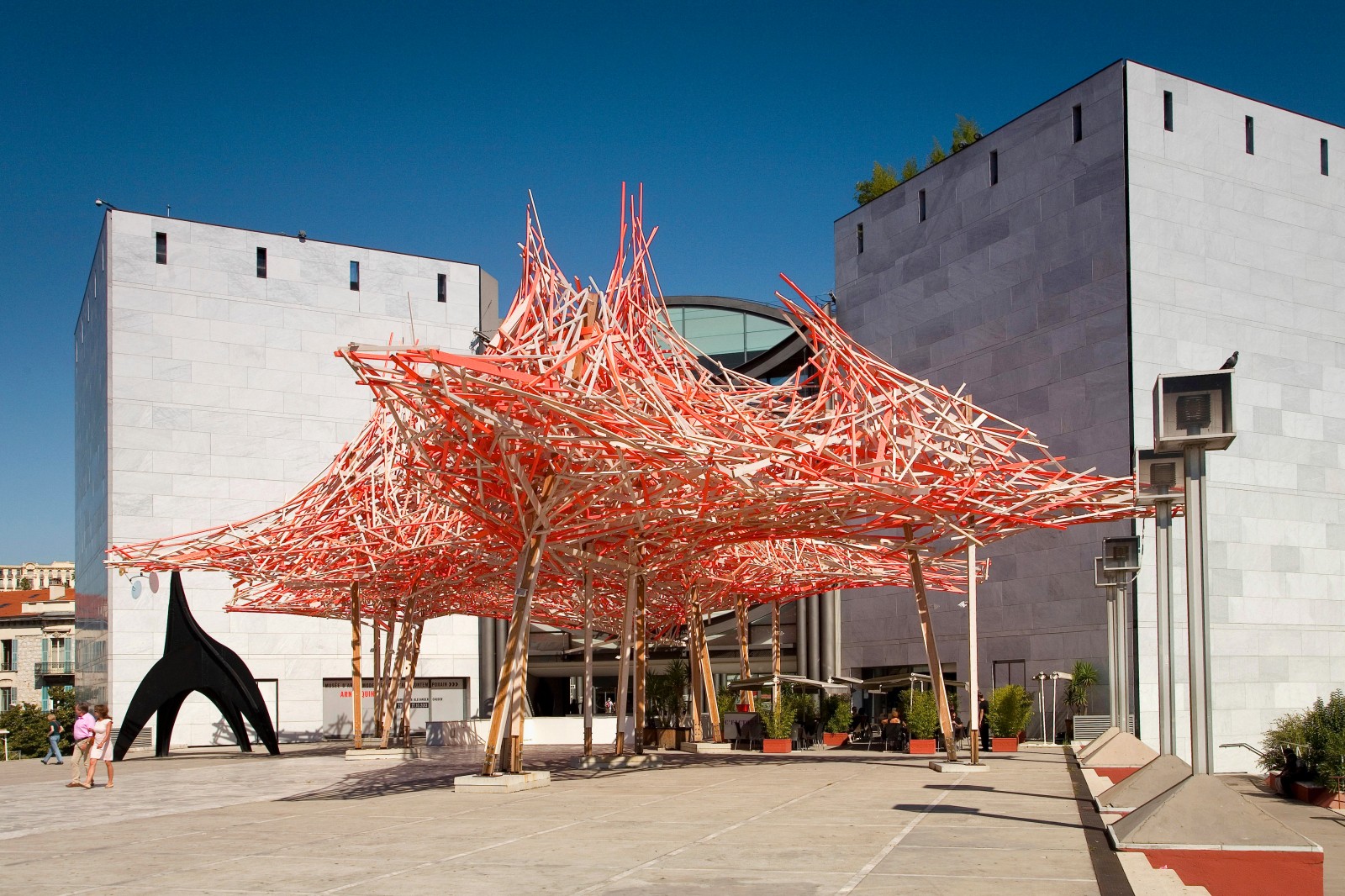The image showcases a striking outdoor art installation in front of a modern, angular building with sleek, white and gray walls and minimal windows. The building's entrance is partially obscured by a sprawling, tent-like sculpture made up of interwoven, reddish-orange and white linear pieces that resemble thatched sticks or oversized woven beach umbrellas. This visually arresting piece is supported by wooden beams that resemble tree trunks, creating a shaded area below. In the foreground, people walk under the sculpture, highlighting its significant height and scale, estimated to be around 25 feet by 25 feet. Nearby, a smaller black metal sculpture reminiscent of Alexander Calder’s work stands in contrast. The scene depicts a sunny day with a clear blue sky, adding a vibrant backdrop to the bustling activity around the building's patio, which features outdoor seating and diners, suggesting it may be a restaurant. A waiter is visible among the diners, contributing to the lively atmosphere of this outdoor space adorned with modern art.